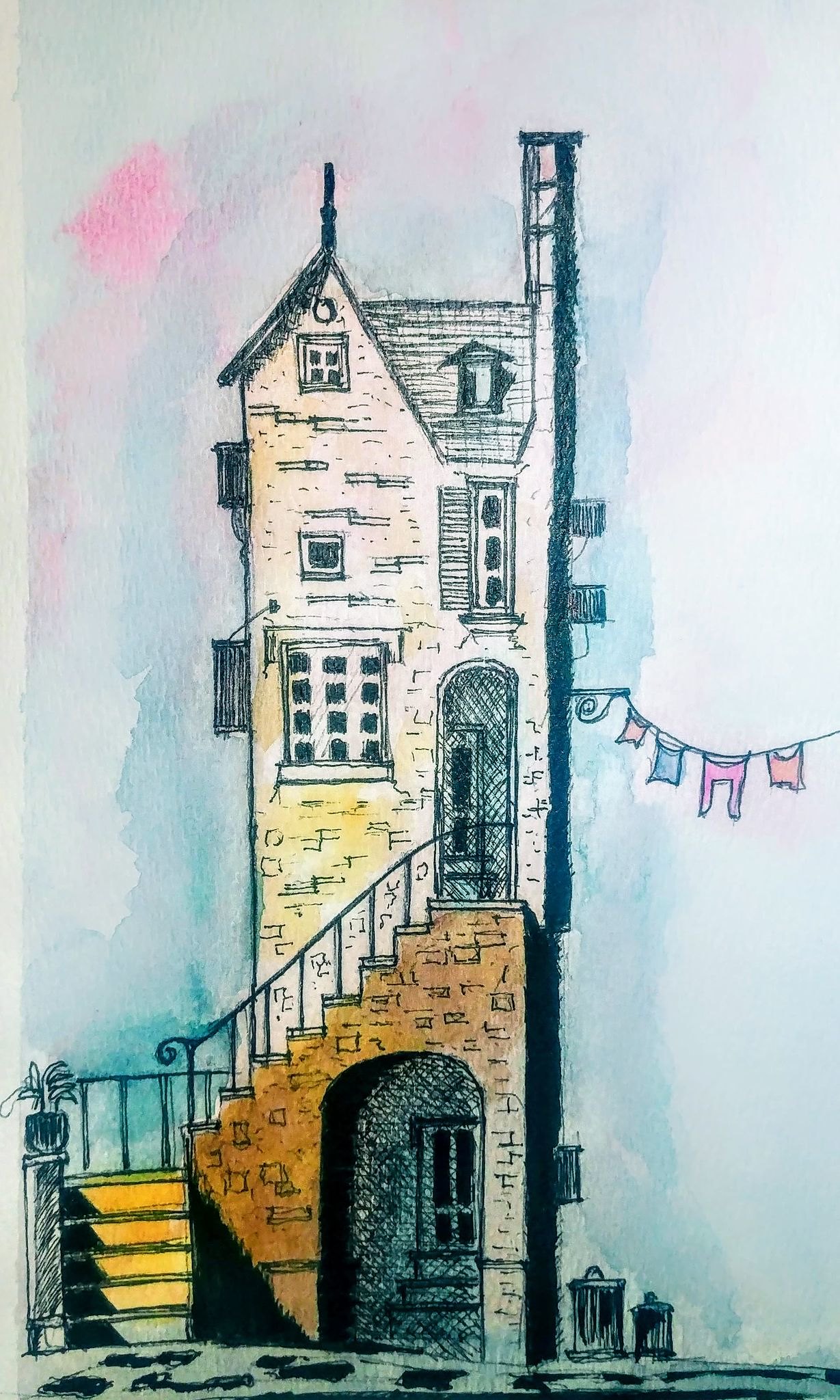This detailed pen and ink drawing, enhanced with watercolor, depicts a narrow, tall European house reminiscent of the one from the French cartoon Madeline. The building, viewed from the side, exhibits three floors and features steep steps turning 90 degrees halfway up. The steps, constructed from brown brick, contrast with the white brick of the house. Beneath the staircase is a round-arched door, and at the top of the steps is another entrance. The building’s façade includes several windows: a single window on the ground floor, another on the first floor, and a narrow second-floor window resembling a traffic light, alongside a smaller one. A tall chimney adorns the roof, which also features an arched gable and a tiny attic dormer window. The surrounding background is beautifully washed with watercolors, blending intense blue aquamarine and pink hues. A clothesline with short cloths adds a touch of daily life, accompanied by two trash cans at the bottom of the stairs.